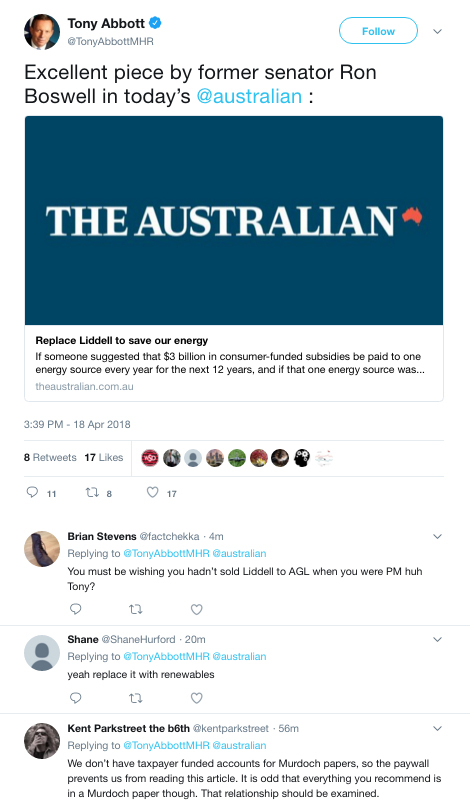**Twitter Post by Tony Abbott MHR**

Profile Information:
- **Username:** Tony Abbott MHR
- **Verification:** Blue circle with a white checkmark
- **Profile Picture:** Close-up of Tony Abbott wearing a coat and tie

Tweet Details:
- **Content:** "Excellent piece by former Senator Ron Boswell in today's The Australian."
- **Image Attached:** 
  - The attached image features a blue box with white font, titled "The Australian" prominently in the middle.
  - Below the title, a blurb reads: "Replace Liddell to save our energy."
  - Additional text states: "If someone suggested three billion in consumer-funded subsidies for one energy source every year for the next 12 years..."

This descriptive caption provides a clear and detailed overview of Tony Abbott's Twitter post, highlighting its relevant elements and content.